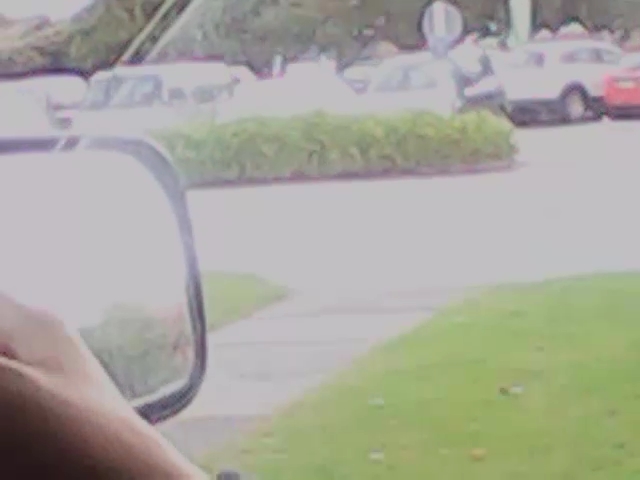A sun-drenched view from inside a car showcases the scene outside through a slightly grimy, closed window, rendering the entire panorama hazy and washed-out from the bright sunlight. The left side of the image prominently features a rear-view mirror, which is partly obscured by the passenger's hand resting on the window ledge. Outside, a manicured green lawn is split by a sidewalk running down the middle, leading into a busy parking lot. A row of well-maintained bushes or hedges creates a natural divider between the lawn and the parking area, beyond which numerous cars are parked, though their details are hard to discern due to the intense brightness. The blending of natural and urban elements makes for a serene yet bustling outdoor environment, partially concealed by the dusty car window.